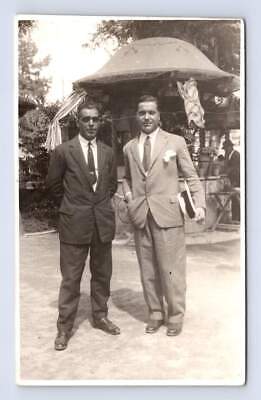This vintage, black-and-white photograph is set within a portrait-oriented layout, featuring a bluish-gray border followed by a white border. At the center of the image, two men are captured in suits. The man on the left is donned in a black suit paired with a black tie and a white shirt. His counterpart on the right wears a lighter suit—possibly khaki or gray—with a white shirt and a matching tie. The man in the lighter suit holds a white hat with a black rim in his left hand and appears to have a white handkerchief in his suit coat pocket. Behind the men is a setting that includes trees and greenery, along with what looks like an outdoor bar with an umbrella-shaped cover and possibly curtains. The ground beneath them seems to be paved or concrete. In the upper left corner of the image, there’s a lighter area hinting at the sky or sunlight.